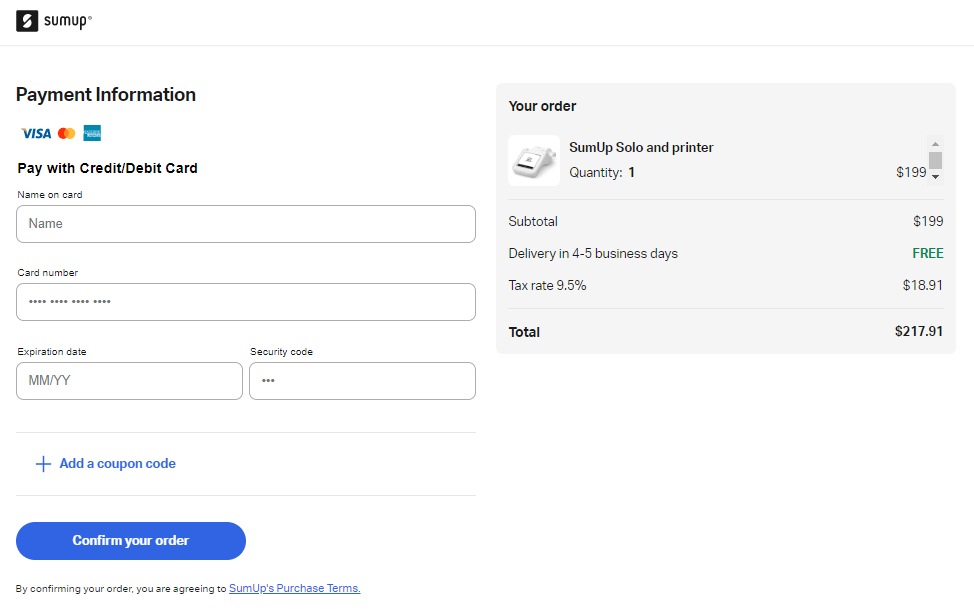The image depicts a payment interface for SUMUP. In the upper left corner, there is the SUMUP logo, featuring a black background with a stylized white “S” formed by two half-circles. Adjacent to this, there is a light gray line with the text "Payment Information."

Below the line, icons for Visa, MasterCard, and American Express are displayed. The section instructs users to "Pay with credit debit card." Fields are available for entering the name on the card, displayed as "Name" in the input box; the card number, represented by four sets of four dots; the expiration date, shown as "MM/YY" in the input field; and the security code, indicated by three dots.

Additionally, there is an option in blue text to "+ Add a coupon code." A prominent blue button labeled "Confirm Your Order" is positioned below, followed by text indicating, “By confirming your order you are agreeing to SUMUP's purchase terms" in blue font.

On the right side of the image, details of the order are provided, showing "Your Order: SUMUP Solo and Printer, Quantity: 1, $199." The subtotal is listed as $199, alongside a notation of "Delivery in 4-5 business days" marked as "FREE" in green. Tax at a rate of 9.5% is calculated to be $18.91, bringing the total amount due to $217.91.